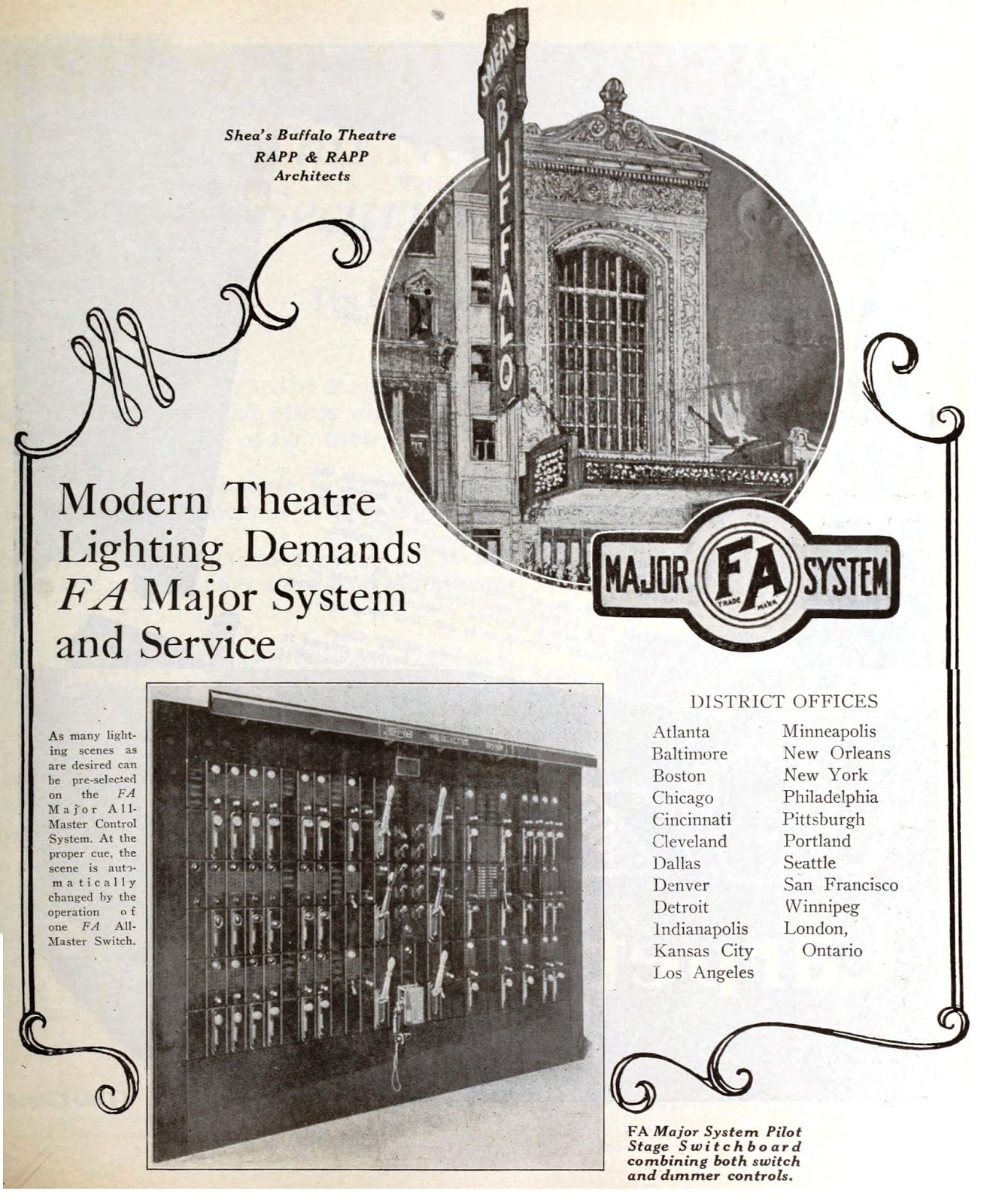This image is an old-style advertisement from a historical newspaper or magazine for the F.A. Major System, a company specializing in theater lighting and electrical services. Dominating the top center is a photograph of the exterior of Shea's Buffalo Theatre, prominently displaying a marquee reading "Buffalo." The left section includes text highlighting "Shea's Buffalo Theatre, Wrap and Wrap Architects," and the slogan "Modern Theatre Lighting Demands F.A. Major System and Service." There is small, unreadable text beneath this, accompanied by an image of a bank of lockers. On the right side, the advertisement lists district offices in various cities across North America, including Atlanta, Baltimore, Boston, Chicago, and many more, extending even to London, Ontario, and Winnipeg. The bottom right corner features a caption stating, "F.A. Major System Pilot Stage Switchboard, combining both switch and dimmer controls," alongside a photo of an antiquated electrical switchboard with numerous levers. Additionally, a logo with "Major F.A. System" encloses the initials "F.A." in a circle, emphasizing the brand's historical significance in theater lighting.